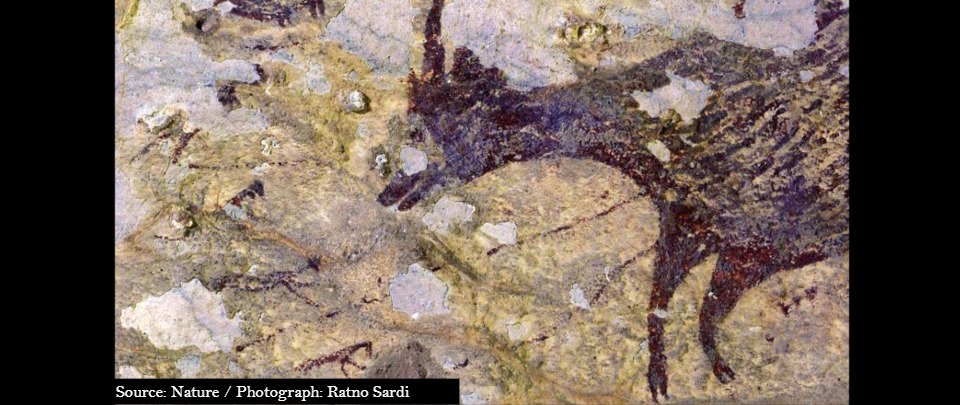The image features an ancient cave painting depicting a large, horned animal resembling a buck or goat, rendered in shades of black and brownish-black. The animal is illustrated facing to the left, with comparatively short front legs and a thicker body, neck, and head. The background showcases the natural texture of the cave, with yellow and gray tones from the surrounding rock. Smaller figures, possibly representing other animals or people, are depicted running towards the larger creature, suggesting movement or a scene of confrontation. The edges of the image are framed with black vertical bars, and a caption at the bottom states, "Source Nature / Photograph Rottno Sardi." The overall appearance of the painting and rock surface suggests antiquity, reminiscent of artifacts found in museums or private collections, and invokes a sense of early human narrative art.